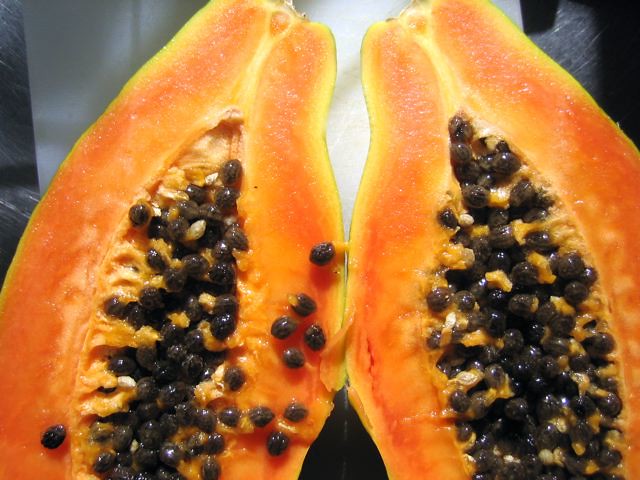This close-up photograph features a papaya that has been cut in half lengthwise, revealing its vibrant, bright orange flesh, which appears juicy and moist. The inner cavity of the fruit is densely packed with small, dark brown seeds, many of which are scattered slightly onto the flesh, likely displaced by the cutting knife. The fruit maintains a symmetrical, oval shape and is showcased against a backdrop that includes a white tissue paper or paper towel. The entire scene is set on a black wooden surface, perhaps a countertop or tabletop, with sunlight subtly illuminating parts of the papaya halves, enhancing the fresh, succulent appearance of the fruit.